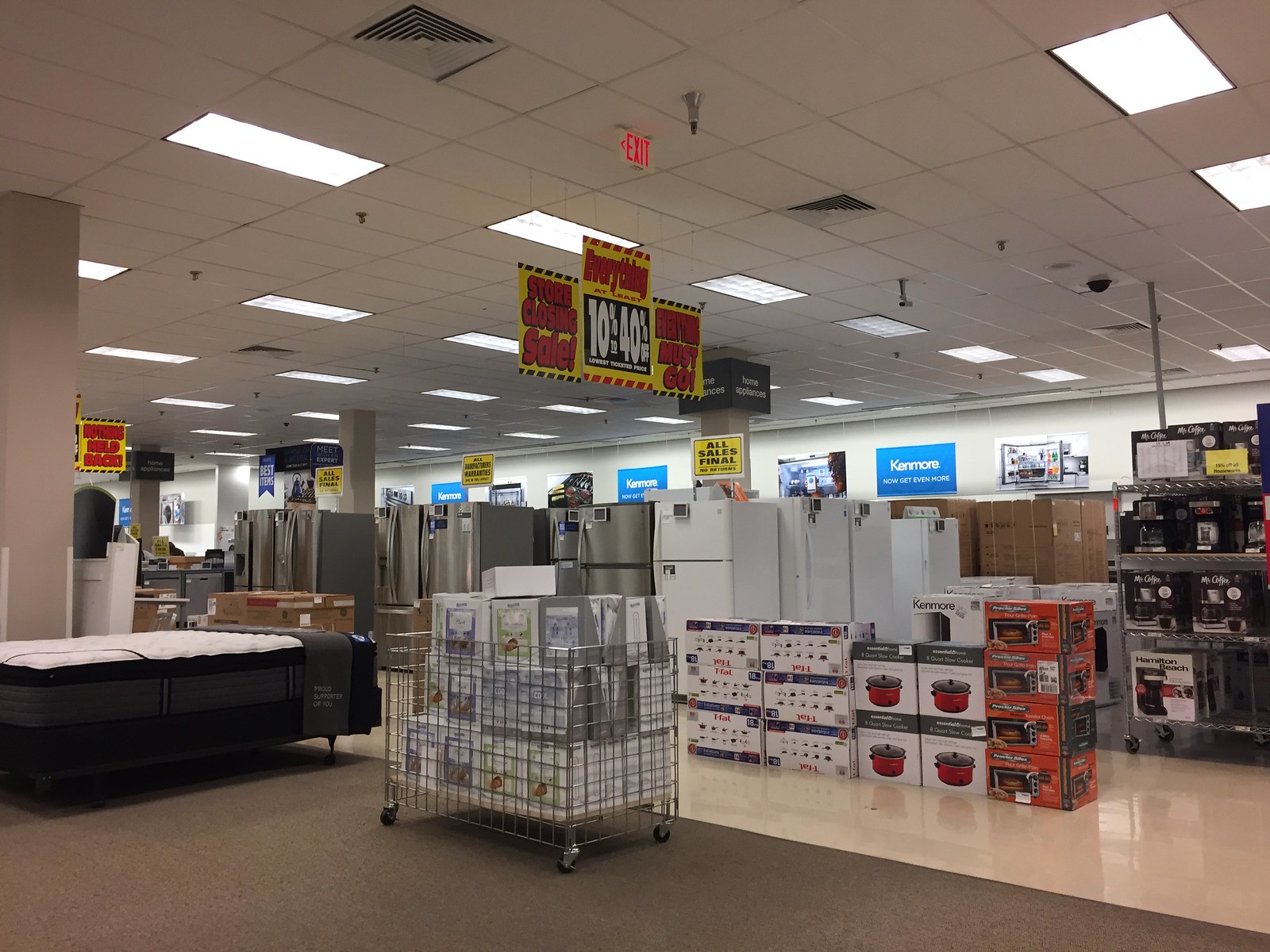The photograph captures an interior view of a department store's appliance section in landscape orientation. The foreground of the image showcases a carpeted area to the left, transitioning to a shiny tiled floor as one moves further into the store. The back wall is adorned with prominent blue signs bearing white lettering that reads "Kenmore, now get even more," accompanied by images above the signs.

Against this back wall stand three to four stainless steel double-doored refrigerators. Just right of these, a row of white refrigerators and refrigerator boxes can be seen. To the extreme right, metal shelves line up, displaying an assortment of countertop appliances. An aisle cutting through the scene contains a display of boxes for brands like T-fal, Crock-Pot, and Kenmore. 

To the right side of the image, a bed is displayed, while more centrally but slightly to the left, a wire cart occupies the carpeted floor space, filled with what appear to be sheets. From the ceiling hangs a yellow sign with red lettering, boldly announcing a "Store Closing Sale," with white lettering advertising discounts ranging from 10% to 40% off. The upper half of the photograph captures an acoustic tile paneled ceiling, fitted with rectangular tiles and industrial lights.